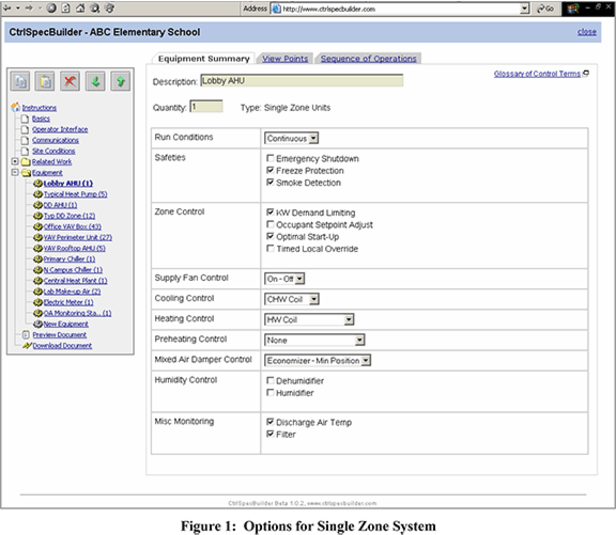This detailed screenshot showcases a web page on the URL "http://www.ctrlspecbuilder.com" featuring the "CTRL SPEC BUILDER" for ABC Elementary School. The webpage header includes the site address and a prominent banner titled "CTRL SPEC BUILDER ABC ELEMENTARY SCHOOL CLOSE."

To the left, a vertical menu lists multiple navigation options: Instructions, Basics, Operator Interface, Communications, Site Conditions, Related Work, Equipment, Lobby AHU, Typical Heat Pump, DD AHU, TYP, DD Zone, Office, VAV Box, VAV Perimeter Link, VAV Rooftop AHU, Primary Chiller, End Campus Chiller, Central Heat Plant, Lab Makeup Air, Electric Meter, OA Monitoring, New Equipment, Preview Document, and Download Document.

On the right side, the "Equipment Summary" section is selected, presenting various equipment and system details:
- **Viewpoint**
- **Sequence of Operations**
- **Description**
- **Lobby AHU**
- **Glossary of Control Terms**

Several attributes and their statuses are listed with some being checked and others not:
- **Quantity:** 1
- **Type:** Single Zone Units
- **Run Conditions:** Continuous
- **Safeties:** Emergency Shutdown (Unchecked), Freeze Protection (Checked), Smoke Detection (Checked)
- **Zone Control**
- **KW Demand Limiting:** Checked
- **Occupant Setpoint Adjust:** Unchecked
- **Optimal Startup:** Checked
- **Time to Local Override**
- **Supply Fan:**
  - **Control:** Central
  - **On/Off:** Off
- **Cooling Control:** CHW Coil
- **Heating Control:** HW Coil
- **Preheating Control:** None
- **Mixed Air Damper Control:** Economizer Min Position
- **Humidity Control:**
  - **Dehumidifier**
  - **Humidifier**
- **Miscellaneous Monitoring:**
  - **Discharge Air Temp:** Checked
  - **Filter:** Checked

At the bottom of the image, it reads "Figure 1, Options for Single Zone System."